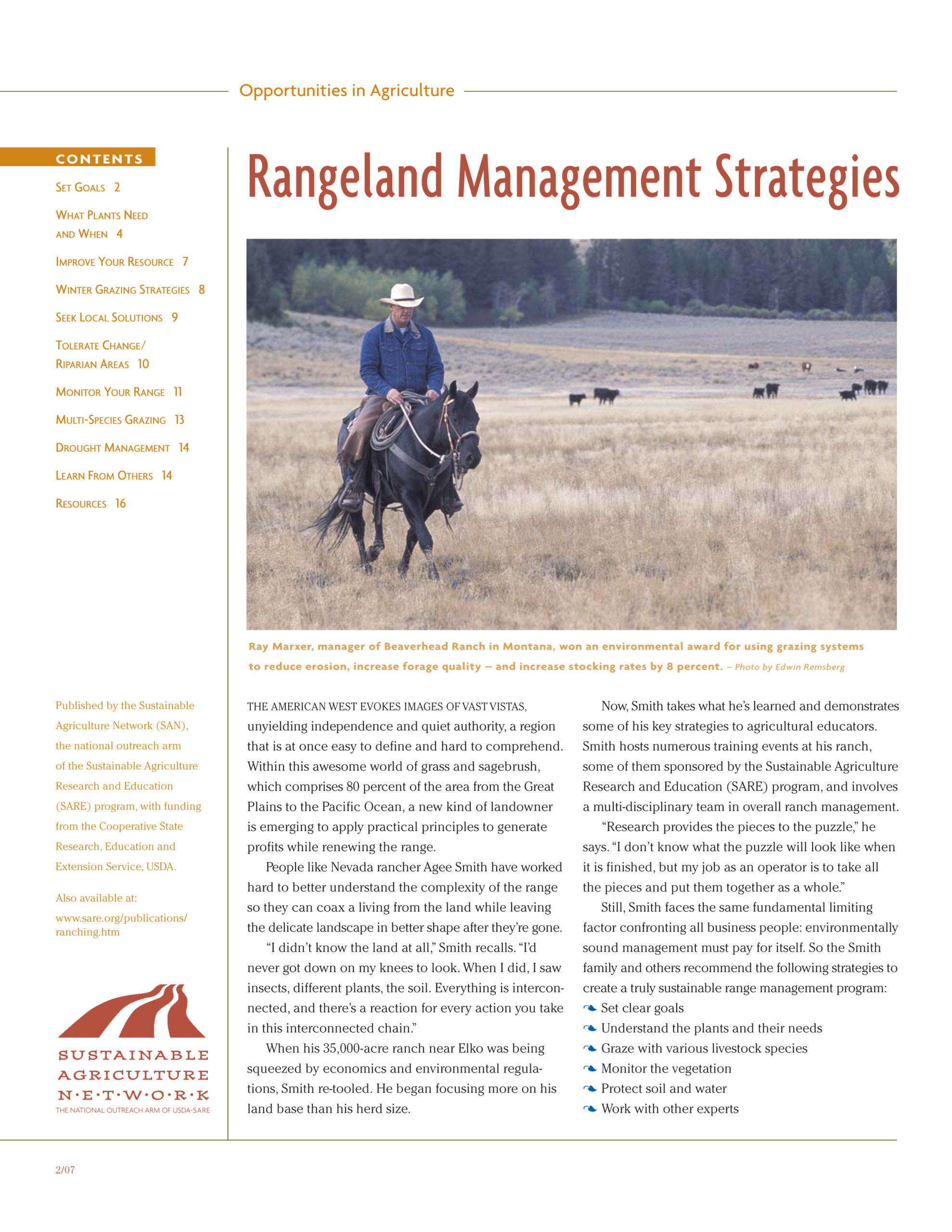The image is a screenshot from an online article in the Sustainable Agriculture Network magazine, appearing under the Opportunities in Agriculture section. The main feature is an article titled "Rangeland Management Strategies," which discusses various grazing techniques. The centerpiece of the article is a photograph of a man riding a dark-colored horse in a field of dry, brown grass, suggesting it might be fall or winter. The rider, identified as Ray Markser, manager of Beaverhead Ranch in Montana, is dressed in a white cowboy hat, a blue long-sleeved shirt or jacket, possibly with a brown collar, and chaps. He holds the reins and has some rope tied up on the saddle. In the background, there are grazing cattle and distant evergreen trees. The page features a yellow table of contents on the left, listing topics like "Set Goals," "Winter Grazing Strategies," and "Drought Management." At the bottom left, there's an orange logo depicting a road, alongside the magazine's name, "Sustainable Agriculture Network." The article praises Markser for using innovative grazing systems that have improved forage quality and increased stocking rates by 8%.